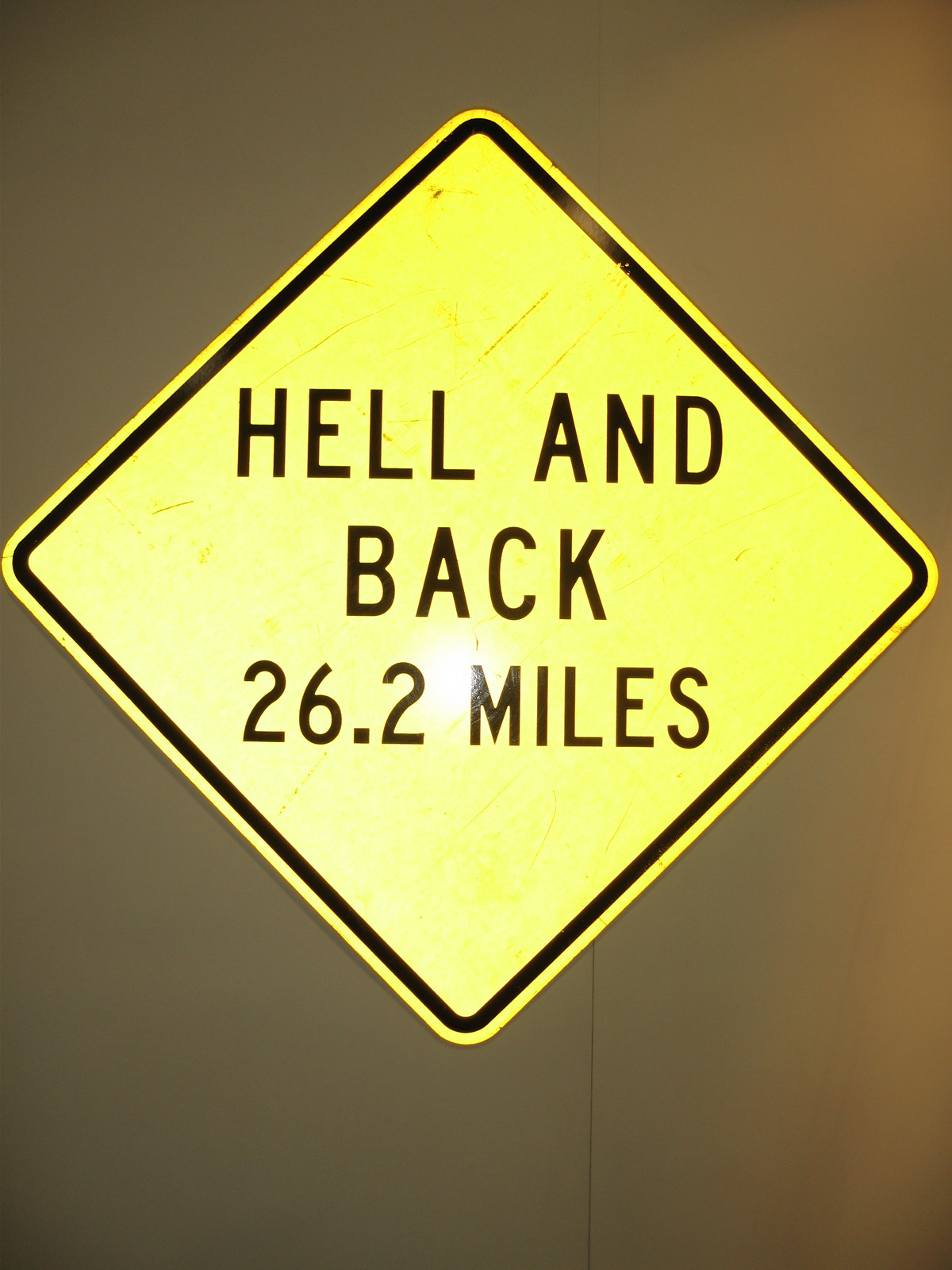**Descriptive Caption:**

A diamond-shaped street sign is prominently displayed against a textured wall with shades of brown and orange, creating a warm, earthy backdrop. The photograph is captured in portrait orientation, effectively centering the sign at the top. The sign is entirely yellow with a thin black border. In the center, bold black capital letters span three lines: the first line reads "HELL," the second line says "BACK," and the third line indicates "26.2 MILES." A distinct glare is visible on the sign, located below the word "BACK" and between the numbers "26.2" and the letter "M" in "MILES," possibly caused by a flash. The sign occupies roughly the top four-fifths of the image, while the bottom fifth is merely the continuation of the blank wall, lending an uncluttered, focused composition.